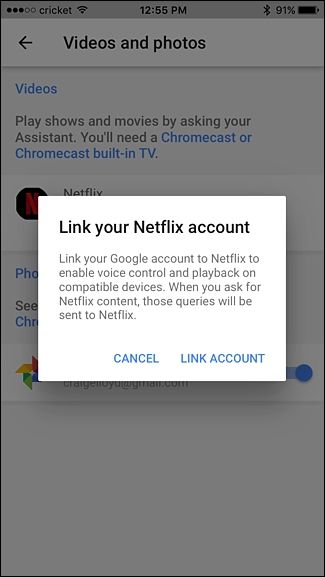Screenshot of a mobile device displaying the Cricut wireless service at 12:55 p.m. with 91% battery, likely from an Android device. The main screen shows a menu titled "Video and Photos" within a larger box. Beneath the main heading, the menu further breaks down into sub-sections for "Videos," "Photos," and other possible options like "Play shows and movies" with a note indicating that Chromecast or a Chromecast-built-in TV is required.

Visible icons on the screen include the Netflix logo with the accompanying text partially obscured by another box. This overlaying box contains the message: "Link Netflix account. Link your Google account to Netflix to enable voice control and playback on compatible devices. When you ask for Netflix content, those queries will be sent to Netflix." Below this message, users are given the options to either cancel the linking process or proceed with linking accounts.

The underlying text, partially covered by the overlay, includes fragments like "ph o" and "CCH" while a portion of the Google logo is visible. To the far right of this, there is a toggle switch that can be turned on or off.